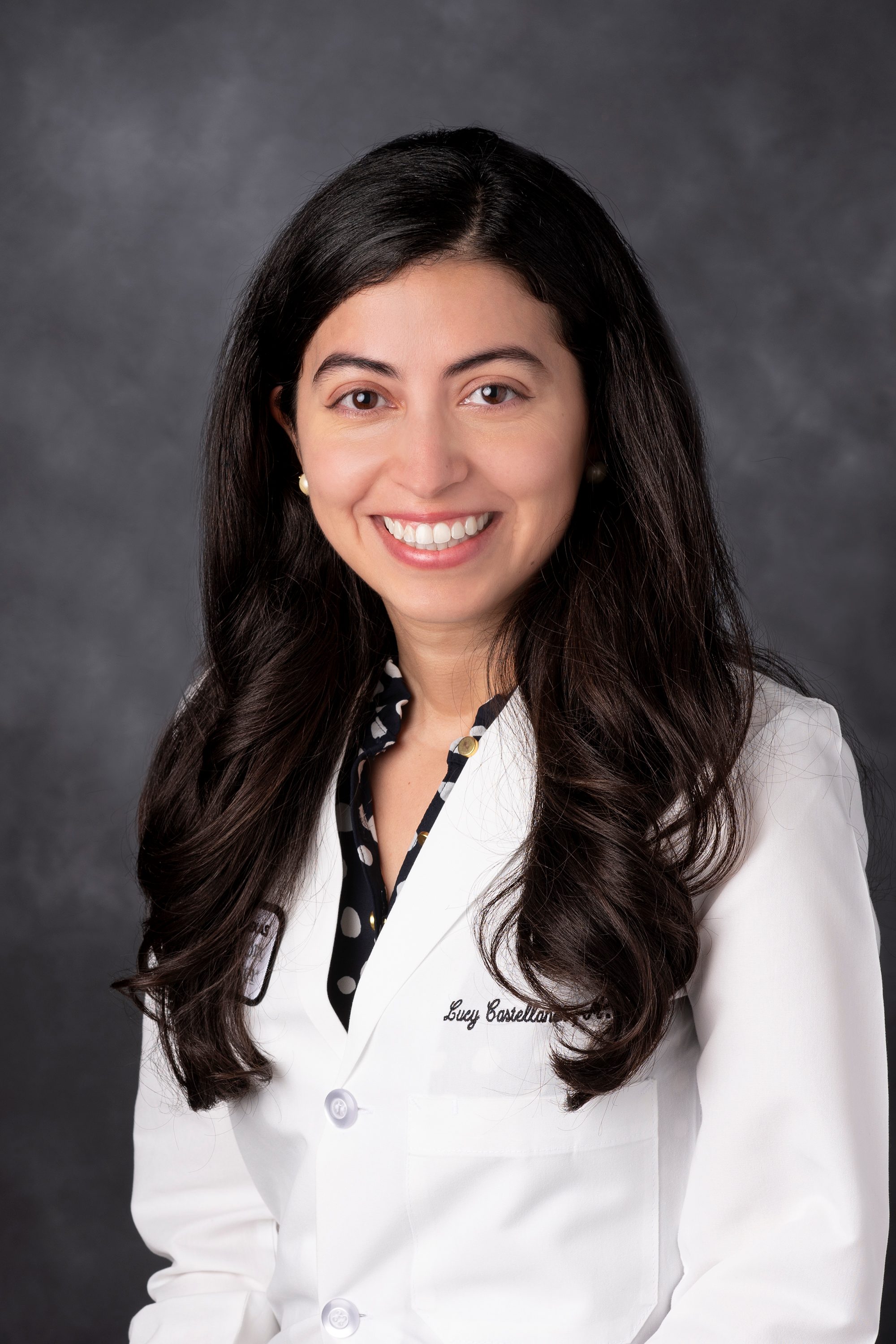In this image, there is a young woman with long, dark brown hair, styled in gentle waves, wearing white earrings. She's dressed in a white medical lab coat with her first name, "Lucy," visible on the right breast pocket, though her last name is obscured by her hair. Underneath her coat, she dons a black and white polka dot blouse with a collar, contributing to a professional appearance. Her features include a round face, almond-shaped brown eyes, and dark, full eyebrows. She is smiling broadly, showing both her top and bottom teeth. The coat also has fine lettering on the left breast pocket, and a sewn patch partially hidden under her hair on the left side. The background is a neutral gray, featuring a mix of darker and lighter shades, giving it a subtle, blurred effect. This polished and professional portrait is likely intended for a platform like LinkedIn or a medical office's website.